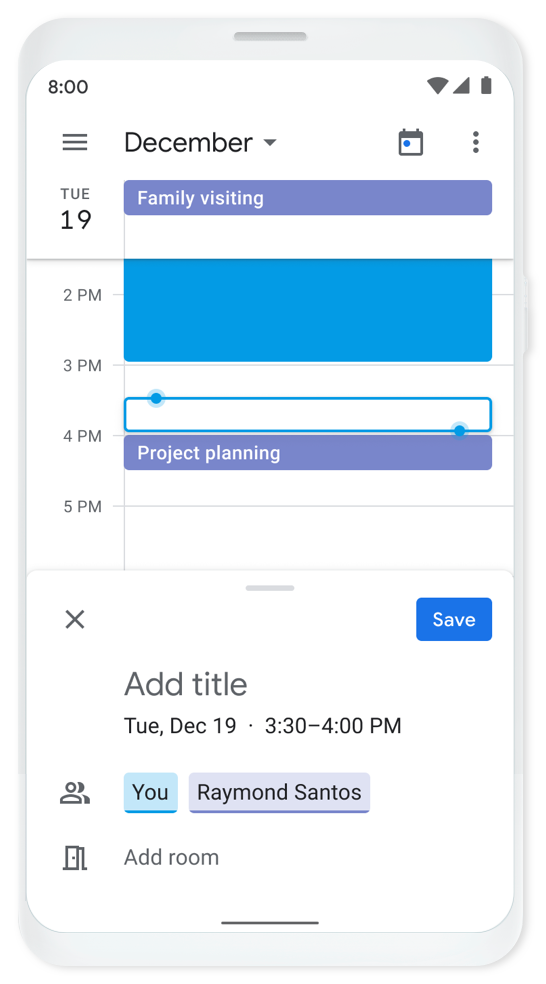A screenshot of a phone screen in a light gray frame displaying a calendar or planner app. At the top of the screen, the current month, "December," is visible along with a drop-down arrow for month selection. To the left, there's a menu icon consisting of three horizontal bars; to the right, a calendar icon and three vertical dots indicating additional settings. Below the header, the date is prominently displayed as "Tuesday 19." 

On the left side, a time sidebar lists hourly slots from 2 PM to 5 PM. A thick blue bar from 2 PM to 3 PM is labeled "Family Visiting." Following this, an empty box appears between 3:30 PM and 4 PM. Lastly, under the 4 PM slot, a purplish-blue bar indicates a "Project Planning" session.

Overall, the screen is neatly organized with color-coded activities and time slots for easy reference.